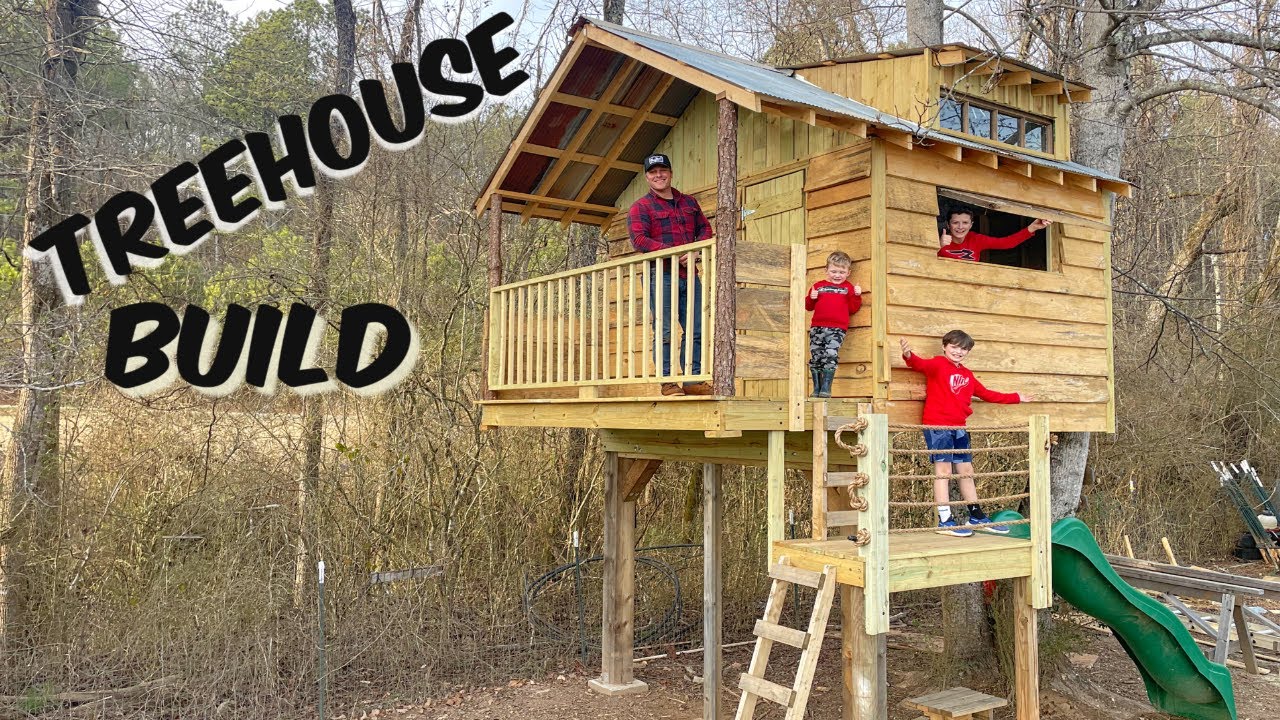This image appears to be an advertisement for a treehouse, prominently featuring bold black bubble letters outlined in white that read "Treehouse Built." Set in what seems to be a family's wooded backyard during winter, the scene showcases a wooden treehouse elevated on stilts. Surrounding the treehouse are leafless, barren trees and a brown field, suggesting the winter season.

The treehouse itself has multiple levels: the first level includes a small platform accessed by a ladder, where a little boy in a red sweater stands. This level also features a green plastic slide extending from it. Another ladder leads up to the second level, which consists of a small enclosed area with windows and a patio secured by a railing. On this second level, a child in a red hoodie peeks out from an open window, while another child in similar attire stands on the porch. Also on the porch is an adult, likely the father or builder, dressed in a red and black flannel shirt, jeans, and a hat, proudly overseeing the scene.

Additional details include ropes around the perimeter of the first level to prevent falls and a tin roof covering the main structure. The overall impression is one of familial accomplishment and pride, highlighted by the smiles and engaged demeanor of the children and their dad.